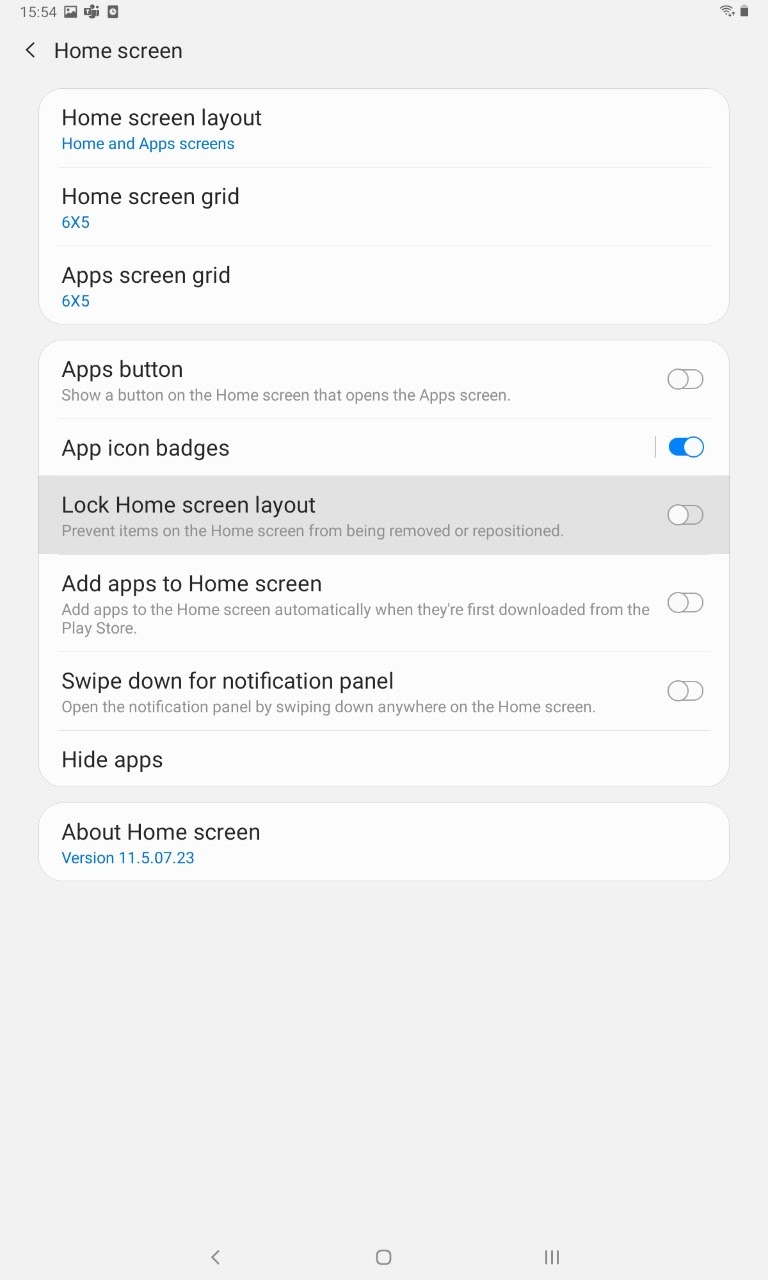This screenshot captures the settings interface of a mobile phone, displayed on a gray background. In the upper left corner, detailed status icons are shown, indicating the current time as 15:54. Alongside the time, there are three icons: a photo icon, a group of people icon, and a square with a circle icon. The upper right corner features the Wi-Fi signal icon and the battery level icon, providing additional status information.

Directly below the status bar, the header reads "Home Screen" in black text, with a left-pointing arrow adjacent to it. The primary settings section consists of a white rectangle divided into three segments by thin black lines. The first segment is titled "Home Screen Layout" in black text, with an option named "Home and Apps Screens" displayed in blue text below it. The second segment is labeled "Home Screen Grid" in black text, followed by the configuration "6x5" in blue text. Similarly, the third segment is titled "Apps Screen Grid" in black text, with "6x5" shown in blue text underneath.

Beneath these segments is another white rectangle divided into six sections. The top section is labeled "Apps Button," with a description below that reads, "Show a button on the Home screen that opens the App screen." To the right of this description is a toggle switch, which is currently in the off position.